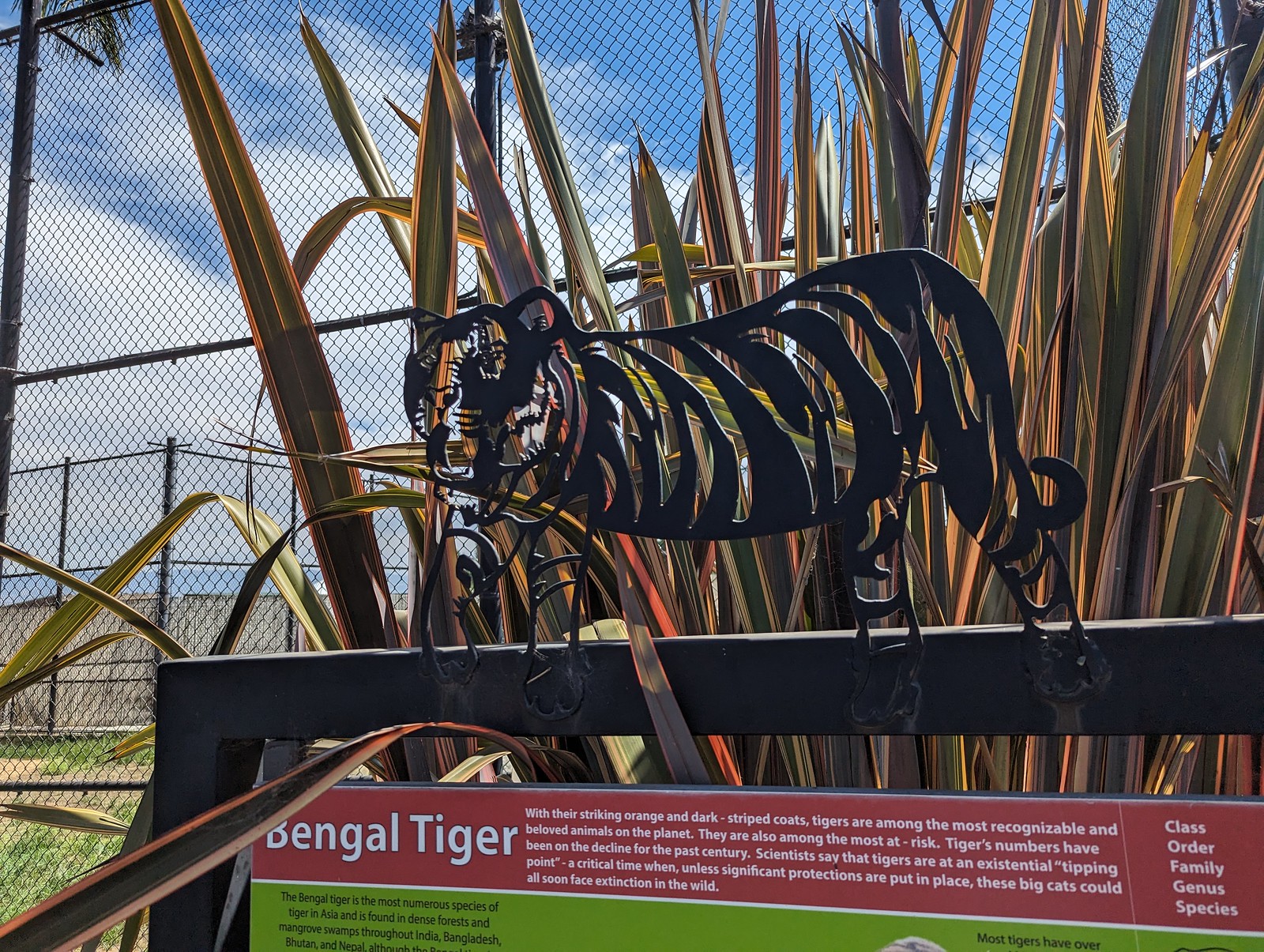The image shows a detailed, artistic metal carving of a Bengal tiger silhouetted against a bright, sunny sky with a few scattered clouds. The tiger's outline and stripes are intricately cut out, leaving open spaces where its striped coat would be. This metal artwork is attached to a U-shaped post composed of horizontal and vertical bars. Below the carving is a large informational sign with a red background and white text that reads, "Bengal Tiger: With their striking orange and dark striped coats, tigers are among the most recognizable and beloved animals on the planet. They are also among the most at risk. Tigers' numbers have been on the decline for the past century. Scientists say that tigers are at an existential tipping point, a critical time when, unless significant protections are put in place, these big cats could soon face extinction in the wild." Tall palm fronds and bamboo stalks provide a lush backdrop, along with a series of chain-link and chicken wire fences that suggest the perimeter of a tiger enclosure, likely at a zoo. The ground is speckled with patches of green grass and brown dirt, adding to the natural setting. Other partially visible details on the sign include taxonomic classifications in white text and a green section with additional information obscured by the image’s framing.